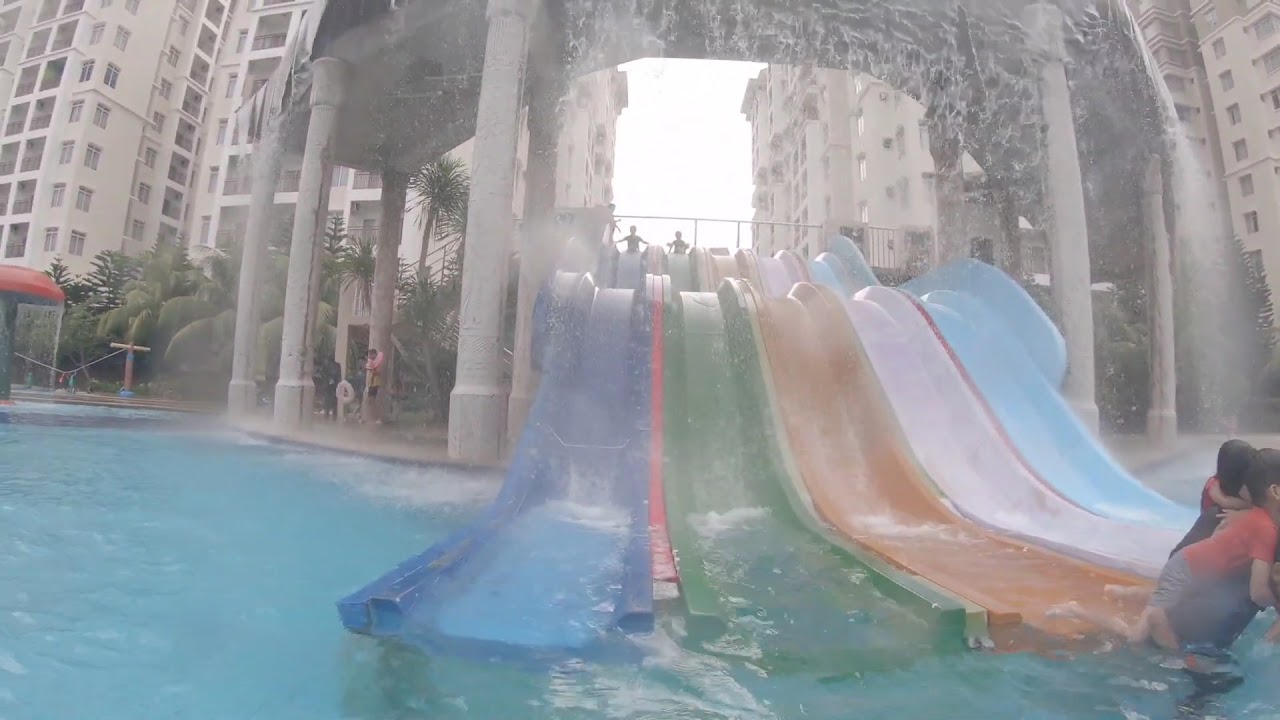This vibrant photograph captures the excitement of a hotel water park, likely resembling the Atlantis in Paradise Island, Bahamas. The scene is dominated by five colorful water slides—blue, green, red, pink, and light blue—that start under a small pavilion, where water cascades down over the slides from an archway, creating a playful waterfall effect as they descend into a turquoise pool. The slides exhibit a dynamic suspension between the architecture and nature; lush trees and a little garden flourish to the left of the pool, which is itself encircled by the hotel’s tall, multi-floored, yellowish brick buildings. Two silhouetted figures, backlit by the sun, await their ride at the top of the slides in the distance, and two kids are seen emerging from the water slide in the bottom right corner, adding a lively human element to the vibrant atmosphere.